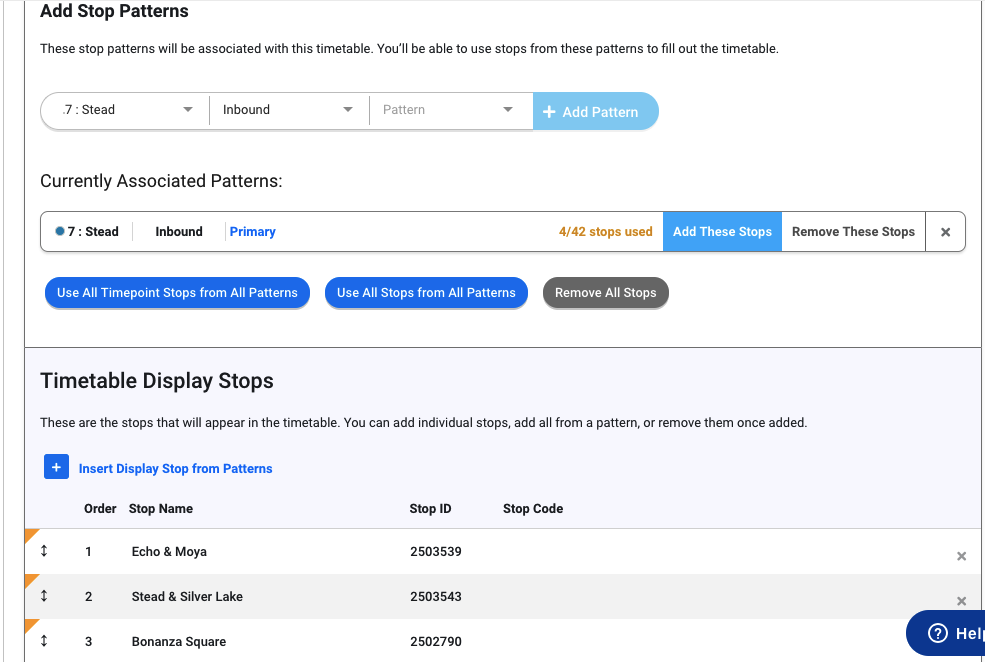This image is a screenshot taken from a website interface for managing delivery service timetables. The top left-hand corner features a title that reads "Add Stop Patterns." Below this title, there's an instructional text explaining that the stop patterns will be associated with the timetable, allowing users to utilize these stops for scheduling deliveries.

In the center of the screenshot, there's a section labeled "Currently Associated Patterns," which offers various options such as "Use All Time Stops from All Patterns" and "Remove All Stops." This section provides tools for managing the stops that appear on the timetable.

At the bottom of the image, three distinct stop names are listed alongside their corresponding IDs. These stops are named:
1. Echo and Moa
2. Stead and Silver Lake
3. Bonanza Square

The interface has a clean, white background with black text, making the information clear and readable. This appears to be an administrative panel for organizing and editing delivery routes and schedules.